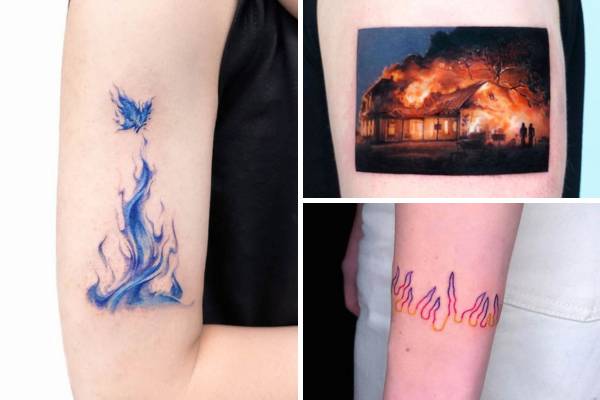The image showcases three juxtaposed photographs of tattoos on different arms. The largest photo on the left side depicts a tattoo on a thin, long, pale upper arm of a blue flame extending upwards, from which a blue ember or butterfly seems to be emerging. On the top right, there’s a hyper-realistic tattoo of a house engulfed in flames, with two silhouetted figures standing in front of it, seemingly witnessing the inferno. Below this, the final photograph features a tattoo that encircles another arm, depicting stylized flames or potentially upside-down icicles, colored in shades of purple, pink, and orange.